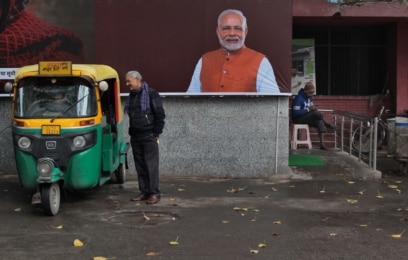This image captures a bustling scene in an Indian parking lot. Dominating the frame, a man with a gray beard and hair, dressed in a red vest over a white shirt, appears on a billboard in the background. This portrait, possibly of a notable Indian figure, hints at the setting being India. In the foreground stands a man next to a traditional Indian tuk-tuk, characterized by its green bottom and yellow top, which is a typical motorized three-wheeler taxi seen in the region. The man, wearing a black sweatshirt, black slacks, and brown shoes, is engaged in conversation with the unseen driver of the tuk-tuk. He has a scarf draped around his neck and maintains a slight smile. The parking lot's concrete surface is scattered with dead leaves, and nearby, a bicycle rack is occupied by a bike, next to which another man in a blue sweatshirt sits on a stool. A manhole cover can be seen on the ground, adding to the everyday urban backdrop of the scene.